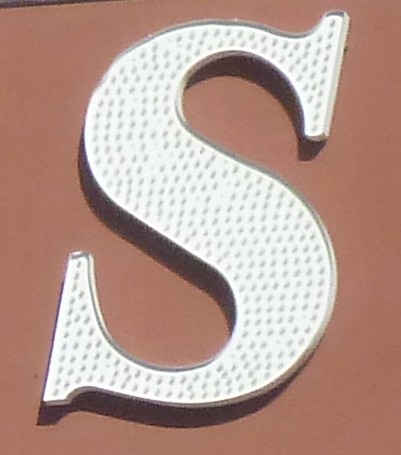A large, white metal letter "S" dominates the center of the image, positioned against a brownish-red background. The "S" appears to be constructed from a sturdy metal and is designed to be illuminated, as it's filled with numerous small light bulbs. These light bulbs suggest that the "S" can light up, adding a vibrant and eye-catching element to its appearance. The base of the "S" casts a reflection onto the surface below, creating a shadowy effect. Notably, in the top left-hand corner of the image, there is a small sliver of black, adding contrast and depth to the overall composition.